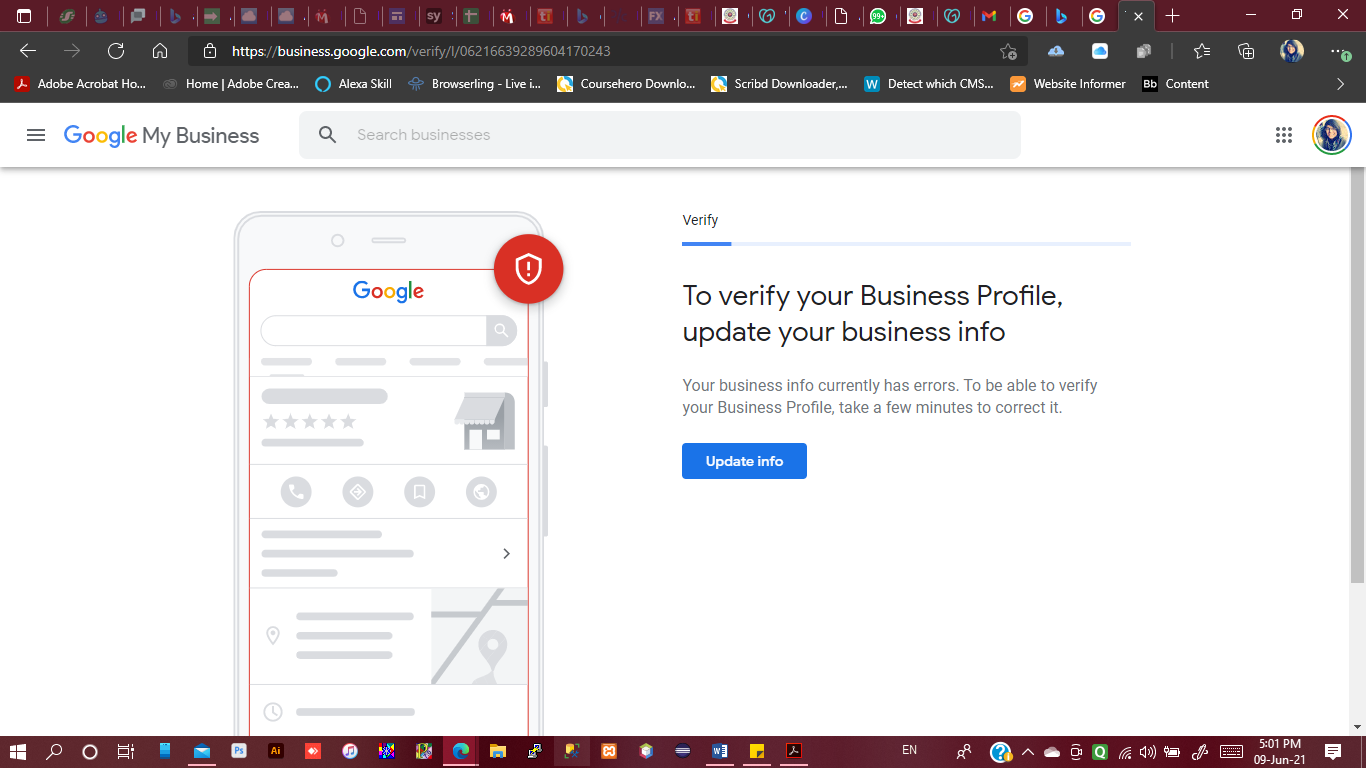The image appears to be a screen capture of a desktop interface. At the top, a thin red-burgundy bar features numerous icons, each varying in color such as white, silver, blue, green, gray, red, orange, purple, teal, gold, and black. Notably, the Google and Adobe logos are present, along with an assortment of other icons.

In the top-right corner, there are typical window control buttons: a minimize button, a maximize/restore button, and a close button.

Below this bar, there is a gray stripe containing navigation elements including back and forward arrows, a refresh icon, a home icon, an address bar with a padlock indicating a secure connection, a star icon for bookmarking, several cloud icons, another star, document icons, and a round profile picture. A three-dot menu is highlighted with a green indicator.

Further down, shortcuts are visible for Adobe Acrobat and other Adobe programs, an Alexa icon, a scribe downloader, and a couple of other miscellaneous icons. A recognizable blue box with a white "W" signifies a Microsoft Word shortcut, alongside an orange box.

In the main content area of the image, "Google My Business" is displayed prominently with a search box beneath it. A gray square is shown alongside a round profile picture. The background is primarily white, featuring a simulated cell phone interface. It reads: "Google" with a red circle and white shield icon, accompanied by a notification stating, "Verify your business profile. Update your business info. Your business info currently has errors. To be able to verify your business profile, please take a few minutes to correct it." A blue "Update Info" button is also present.

At the very bottom, another red-burgundy bar shows a variety of icons, a Windows search bar, and a text bubble icon. The system clock reads 5:01 PM, with the date indicated as June 09, 2021.